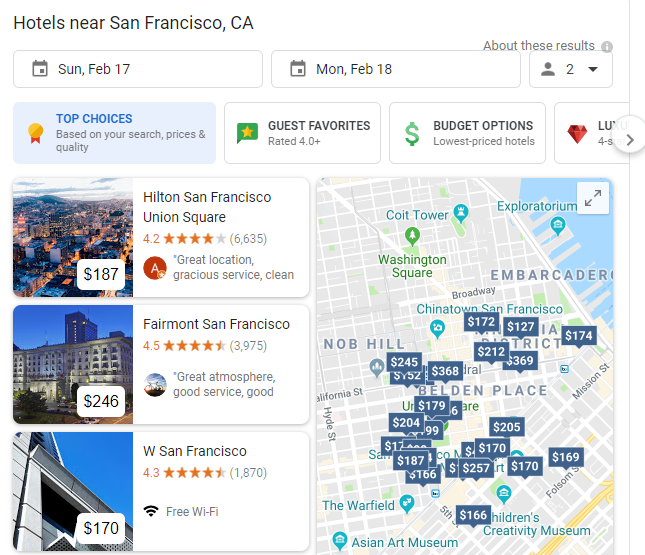A screenshot displaying a search for hotels near San Francisco, CA. The page has a clean white background with several sections aimed at filtering hotel options. At the top, the search query "hotels near San Francisco, CA" is visible, accompanied by a date selector showing "Sun, February 17th to Mon, February 18th" and a gray icon of a person indicating a booking for two guests.

Below the search details, there are categorized filter sections with a gray border:

- **Top Choices**: Highlighted in light blue, features "top choices based on your search prices and quality" with a gold and red ribbon icon.
- **Guest Favorites**: Shows "guest favorites rated 4.0+" with a green icon featuring a gold star.
- **Budget Options**: Lists "lowest price hotels" with a green cash sign.
- **Luxury**: Partial text "LUXU 4 star" with a red ruby icon, text cut off.

The main content features images and details of specific hotels:

1. **Hilton San Francisco Union Square**:
   - City view tinged with hues of orange and blue.
   - Priced at $187 per night.
   - Rated 4.2 stars from 6,635 reviews.
   - Highlighted review: "Great location, gracious service, clean."

2. **Fairmont San Francisco**:
   - Image of a gray multi-story building.
   - Priced at $246 per night.
   - Rated 4.5 stars from 3,975 reviews.
   - Review excerpt: "Great atmosphere, good service, good."

3. **W San Francisco**:
   - Features free Wi-Fi with the Wi-Fi symbol.
   - Priced at $170 per night.
   - Rated 4.3 stars from 1,870 reviews.
   - Image showing white siding on a house against a blue sky.

To the right, a map resembling a Google Maps interface displays part of San Francisco. Several landmarks are marked, including Coit Tower, Washington Square, Knob Hill, Children's Creativity Museum, Asian Art Museum, and The Warfield. The map features teal icons and a mix of white and blue price markers, with some yellow-marked streets. Notably, specific locations like Washington Square have distinct green icons, and there's an expansion arrow for detailed navigation.

The overall layout is user-friendly, providing both visual and textual information to help users make informed decisions about their accommodation in San Francisco.